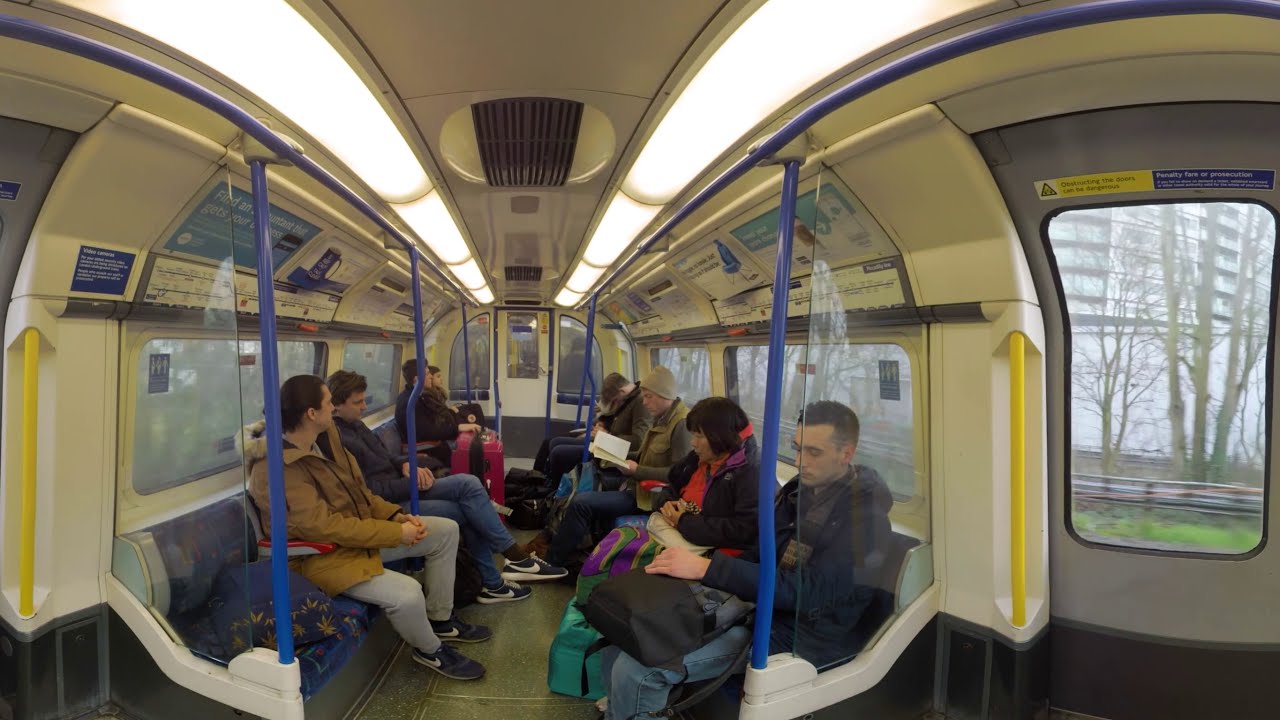A group of middle-aged, ethnically diverse passengers are seated on a modern European train, likely in a city in England, based on the English signage and architecture visible through the windows. The weather outside appears gloomy and gray, with apartment buildings, trees, and the occasional colorful detail in the background. Inside the train, passengers are facing each other on either side of the aisle, all seemingly absorbed in their own activities or quietly waiting for their destination. 

One man with short brown hair is holding a backpack and looking down, while next to him, a woman with short black hair sits with her hands clasped together. Across from her is a man with long brown hair dressed in a brown coat, gray pants, and blue Nikes, and beside him, another man with dark Nike sneakers sits with his legs crossed. Another passenger, wearing a green vest and a hat, is engrossed in reading a book. Towards the back, a man with a pink suitcase sits next to a barely visible woman, while another man, whose head is drooped down as if he's sleeping, rounds out the scene.

The train features blue and yellow handles for standing passengers, although everyone has a seat. Overhead, a small billboard displays various product logos, adding to the modern ambience of the transit system. Despite some appearing displeased or tired, the passengers generally mind their own business, making for a tranquil, if subdued, travel environment.